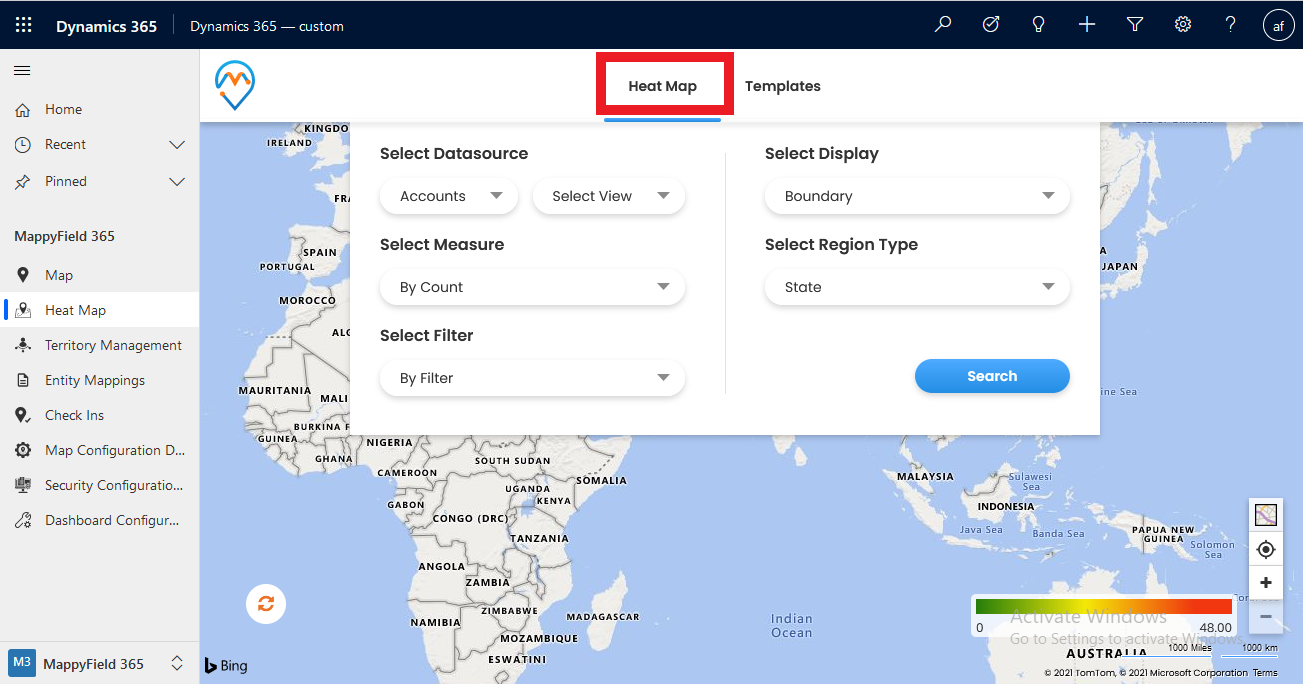Screenshot of a Microsoft Dynamics 365 application interface:

At the top, the black header bar prominently displays "Dynamics 365." To its right, in smaller text, it reads "Dynamics 365 - Custom." The header bar also includes various icons from left to right: a search icon, a check icon, a light bulb icon, a plus icon, a funnel icon, a settings gear icon, a question mark icon, and a circular icon with the initials "AF".

On the left-hand side of the interface, there is a vertical menu column. At the top of this column is a grid of nine dots arranged in a 3x3 configuration. Below the grid, the menu includes the following items:
- Home
- Recent
- Pinned
- MappyField 365
- Map
- Heat Map
- Territory Management
- Entity Mappings
- Check-Ins
- Map Configuration
- Security Configuration
- Dashboard Configuration

To the right of this vertical menu, there is a main content area. This includes a white box outlined in red labeled "Heat Map," indicating its importance. Under this box, there are sections labeled Templates and Category, followed by an overarching section titled "Map."

Overlaying the map area is another box with several selection options:
- Select Data Source
- Select Measure
- Select Filter
- Select Display
- Select Region Type

The detailed layout highlights the structured and feature-rich interface of the Dynamics 365 application, providing users with a variety of tools and configurations at their fingertips.